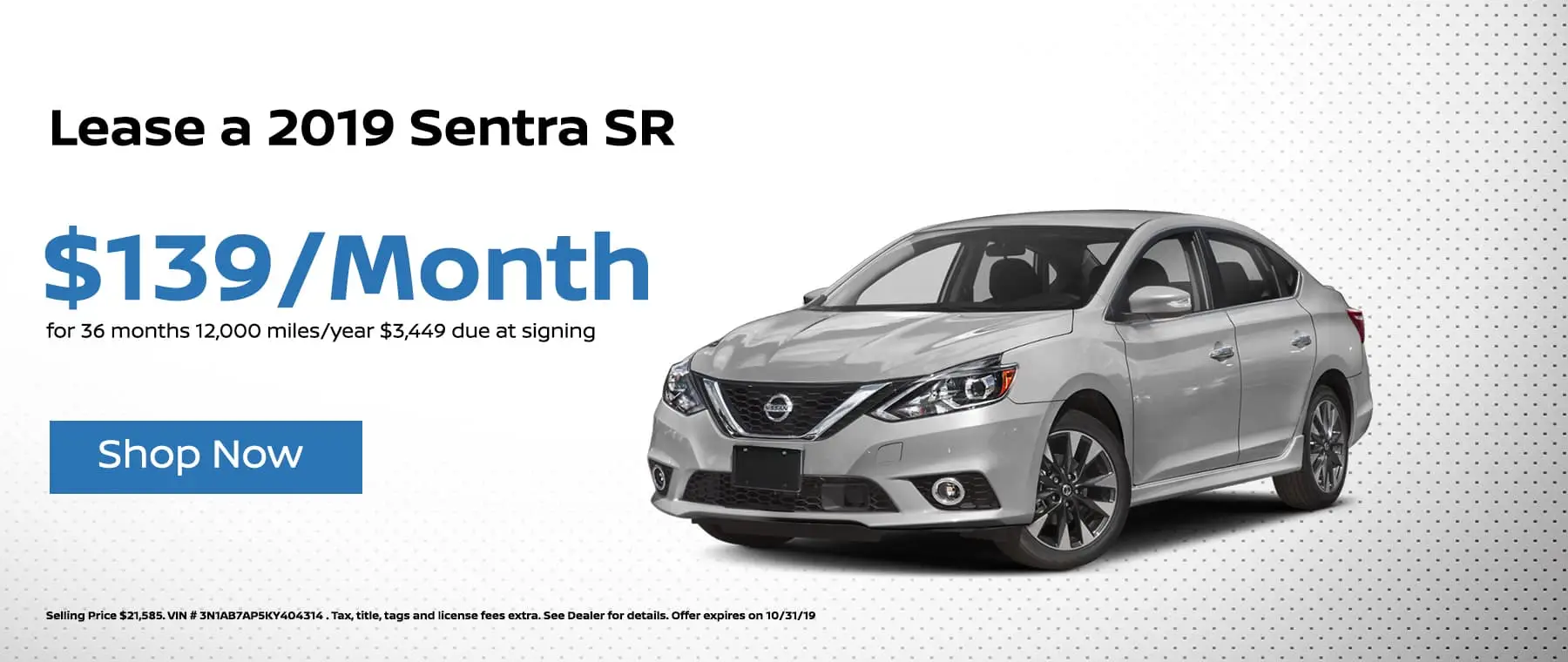The image appears to be an online advertisement for leasing a car. The focal point of the ad is a silver 2019 Nissan Sentra SR positioned towards the right side, diagonally angled to showcase the vehicle's front and left side. The car's design features a black grille with a silver badge, no number plate, a four-door body, and visible seating through the glass. The background is predominantly white, transitioning to gray with a pattern of evenly spaced dots on the right side and bottom of the image.

Text details are prominently displayed on the left side of the image. At the top left, bold black text reads, "Lease a 2019 Sentra SR." Below that in blue text, it states the lease terms: "$139 a month for 36 months, 12,000 miles per year, $3,449 due at signing." Further down, there's a blue rectangular button with white text that says, "Shop Now." Additional details in small black print at the bottom left mention the selling price of $21,585, the VIN number (3N1AB7AP5KY404314), and a note that tax, title, tags, and license fees are extra. It also advises seeing the dealer for details and mentions that the offer expires on 10/31/2019.